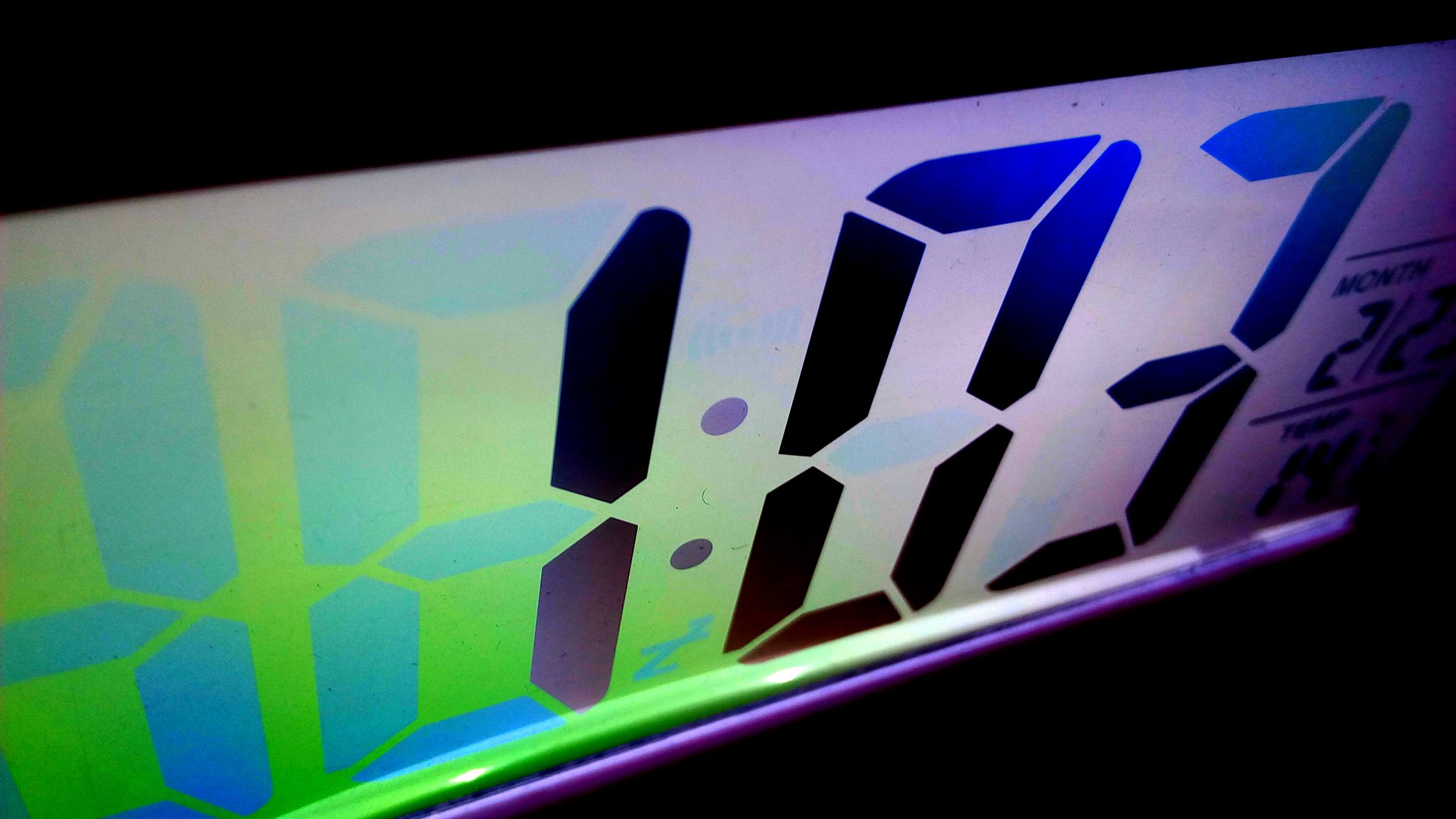The image depicts a close-up of a rectangular digital clock's LCD display set against a jet-black, textureless background. The display details a distinctive glowing effect, with the left side exhibiting a faint green hue and the right side a bluish glow. The primary focus is the time, shown as "1:03" through partially connected dashed lines. To the right, the display indicates the month as "2" before being cut off, preventing further clarity. There is an additional, partially visible readout that seems to say "TEMP" alongside numbers resembling "143" or "14.30," though this part is blurry and ambiguous. The dark setting and the illuminated LCD create a one-dimensional, almost ethereal presentation.